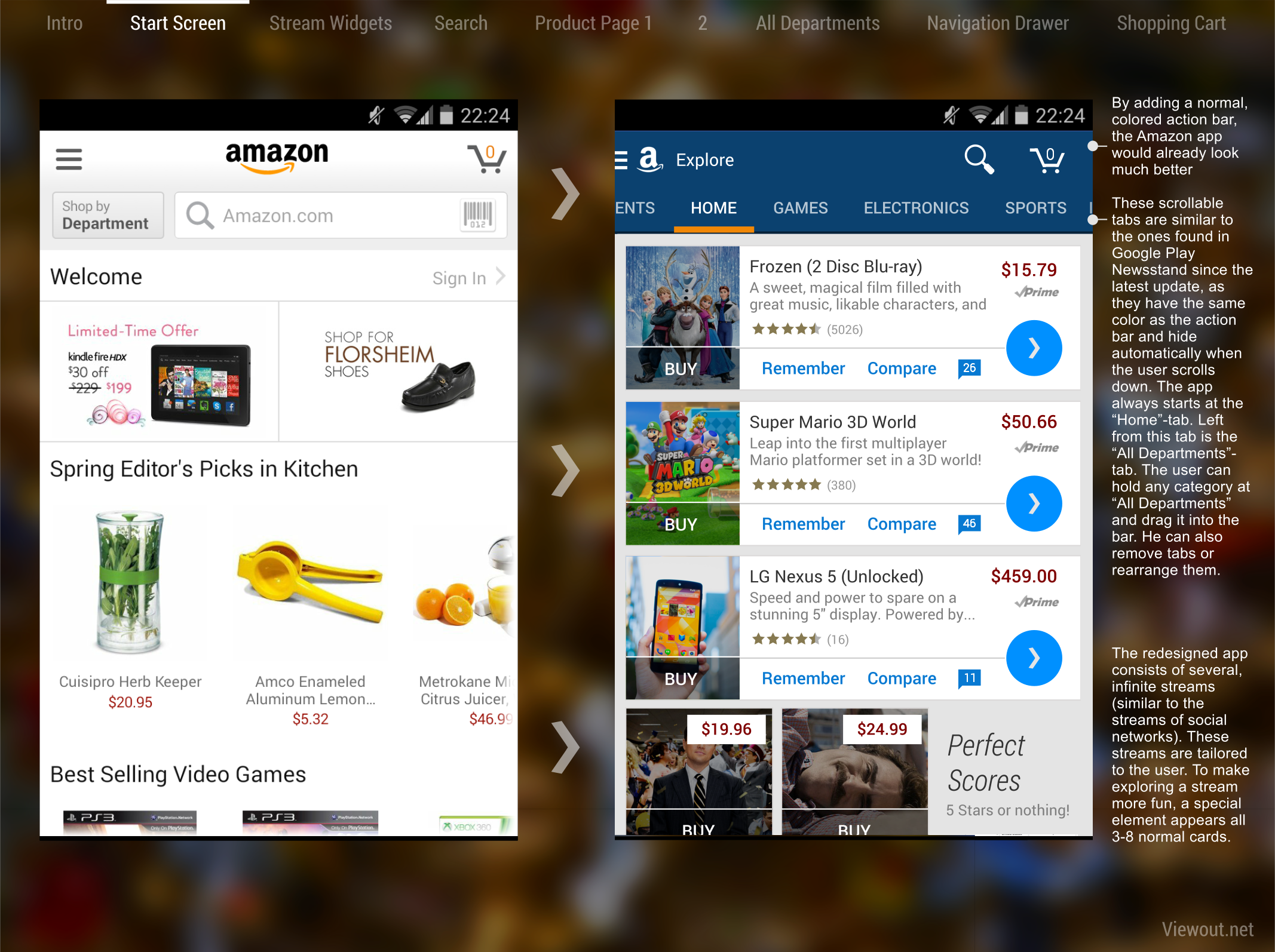An image details a screenshot of a monitor, showcasing elements from the Amazon mobile website interface. The monitor's display has a blurry brown background, with two vertically aligned smartphone screen captures positioned side by side—left and right. Across the top of the monitor, a white navigation menu features labels: Intro, Start Screen (bolded), Stream Widgets, Search, Product Page 1, Product Page 2, All Departments, Navigation Drawer, and Shopping Cart.

### Left Smartphone Screen Capture:
This image displays a typical Amazon webpage with a white background. A black navigation bar sits at the top featuring black cell phone icons and a yellow curved arrow under the Amazon logo. The black shopping cart icon, containing a yellow zero, resides next to a search bar. Beneath this, in black text, it says "Welcome" on the upper left.

* **Products Displayed:**
  * **Limited Time Offer:**
    - Kindle Fire HDX (left)
    - Floor Shime Shoes (right)
  * **Spring Editor’s Picks in the Kitchen:** (Displays three products with pricing)
    - Cuisipro Herb Keeper
    - Amco Enameled Aluminum Lemon (unreadable rest)
    - Metro Cane Citrus Juicer

At the bottom of this screen capture, the section titled "Best Selling Video Games" is partially visible, showing the top of two PS3 game boxes.

### Central Divider:
A number of gray right arrows separate the left and right smartphone images.

### Right Smartphone Screen Capture:
Similar to the left, this image also reveals an Amazon webpage. The top navigation bar includes white icons on the right. Below, a blue banner with white menu labels—Home (highlighted with an orange underline), Games, Electronics, and Sports—is visible. The "currently selected" section under Home shows several product listings.

* **Products Displayed:**
  * **Left Side:**
    - Frozen 2-Disc Blu-ray
    - Super Mario 3D World
    - LG Nexus 5 Unlocked
  * Each product window includes a white "Buy" button at the bottom and a bit of product information above the buy button.
  * An emboldened section in blue offers "Remember" on the left and "Compare" on the right, divided by a gray line.

* **Additional Products:** 
  - Super Mario 3D World repeated
  - LG Nexus 5 Unlocked repeated

* **Bottom Images:**
  * **Left Image:**
    - A man's face covered by a white rectangle that reads "1996" in red, with "Buy" in white at the bottom.
  * **Right Image:**
    - A man's head resting sideways facing the camera, with a white rectangle reading "2499" in red, and "Buy" in white at the bottom.
    - To the right, a section in gray with black text proclaims, "Perfect scores, five stars or nothing."

Finally, several paragraphs of text in white are positioned against the brown background on the far right side of the monitor screen.

This highly detailed visual breakdown intricately describes the captured monitor screenshot exhibiting elements from the Amazon mobile interface.